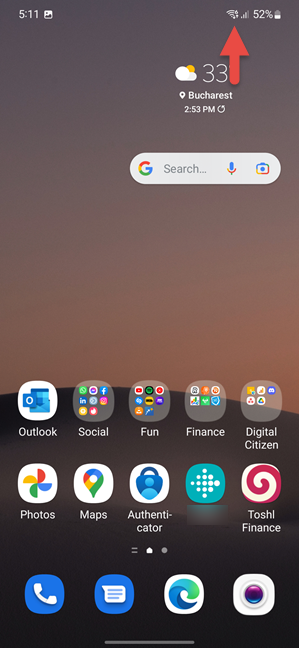This is an image of a smartphone screenshot. In the upper right corner, there are icons indicating Wi-Fi reception and the battery level, which shows 52%. On the upper left, the time is displayed as 5:11. Just below this, to the right, is a weather icon featuring a cloud and a yellow sun, with the temperature 33°C shown in gray text next to a large red upward-pointing arrow. Below the weather information is a map icon alongside the city name "Bucharest" and the local time, 2:53 p.m. Further down, there's a Google search bar featuring the "G" icon for Google, a microphone icon, and a camera icon.